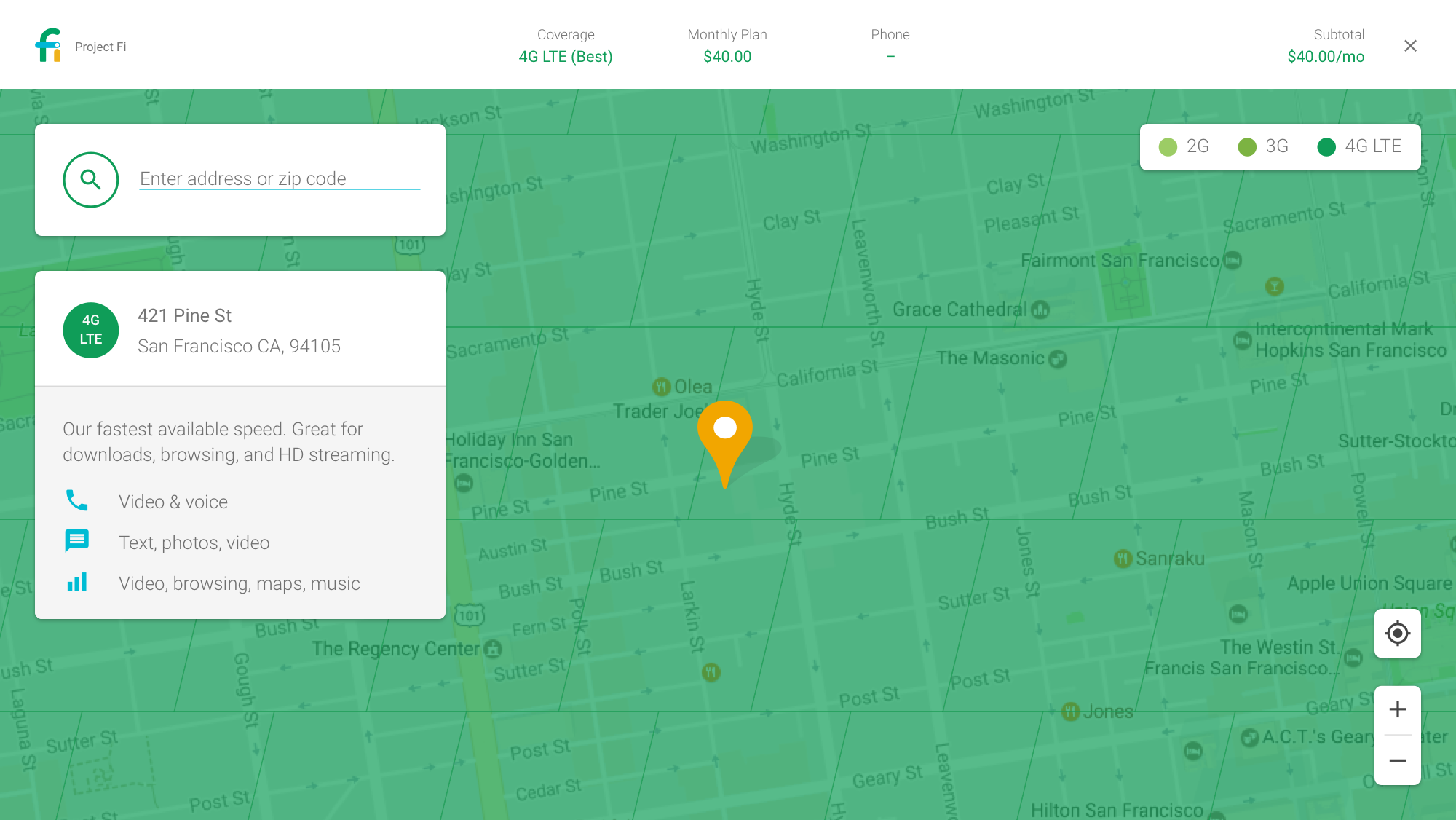The image captures a Project FI plan comparison interface. At the top left, it displays the "Project FI" logo with the text "Coverage" in gray and "4G LTE" in blue, with "best" in parentheses. The monthly plan is highlighted at $40, shown in green text next to a subtotal of $40. A gray 'X' button is visible, presumably to close the interface.

A rounded white rectangle appears prominently on the screen, possibly the search bar. It has the icon of a magnifying glass and text prompting to "Enter address or zip code." Below this, the user has entered "421 Pine Street, San Francisco, CA, 94105."

The coverage information for this location is detailed, indicating that 4G LTE is available and is ideal for activities such as downloads, browsing, and HD streaming. The response goes further to specify that video and voice calls, texting, photo sharing, and music streaming are supported with full signal bars for video, browsing, maps, and music.

To the top right, the image includes a signal indicator bar with "2G, 3G, 4G LTE" highlighted in green. Adjacent to this, there's an apparent tracking location icon with plus and minus buttons below it, likely for zooming in and out.

At the center of the map is a blue and green filter overlay marking the coverage, with a yellow pin and a white dot in its center. Lines are also depicted, likely indicating roads or boundary demarcations.